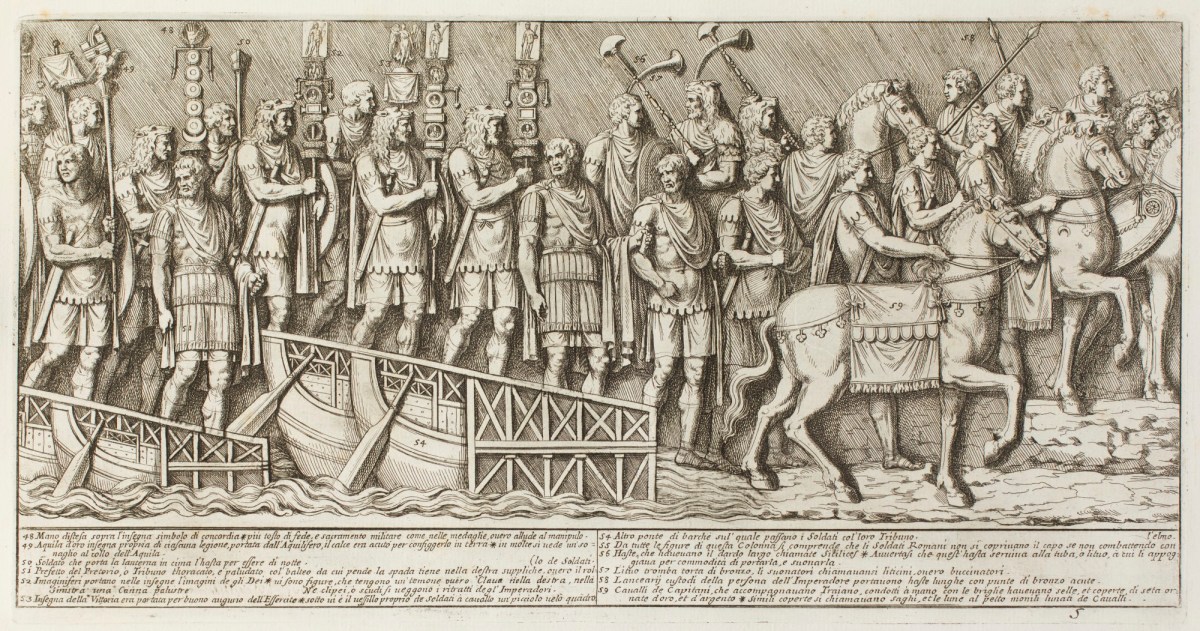The image depicts a detailed grayscale drawing of a Roman legion, characterized by a variety of soldiers in traditional ancient armor and uniforms. These warriors are marching, brandishing swords and spears, and carrying symbols mounted on poles. In the forefront stands a rider astride a horse, likely guiding it or riding it forward. The horse appears suited for chariot use, its front legs mid-stride. Positioned to the right, there are several boats docked in the water, suggesting preparations for a military campaign. Below the scene, written in an aged, italicized font on what seems to be a rolled-out piece of paper, are inscriptions that hint at a historic narrative or declaration. The image is rectangular, twice as wide as it is tall, framing the regimented advance of soldiers towards an impending conflict.